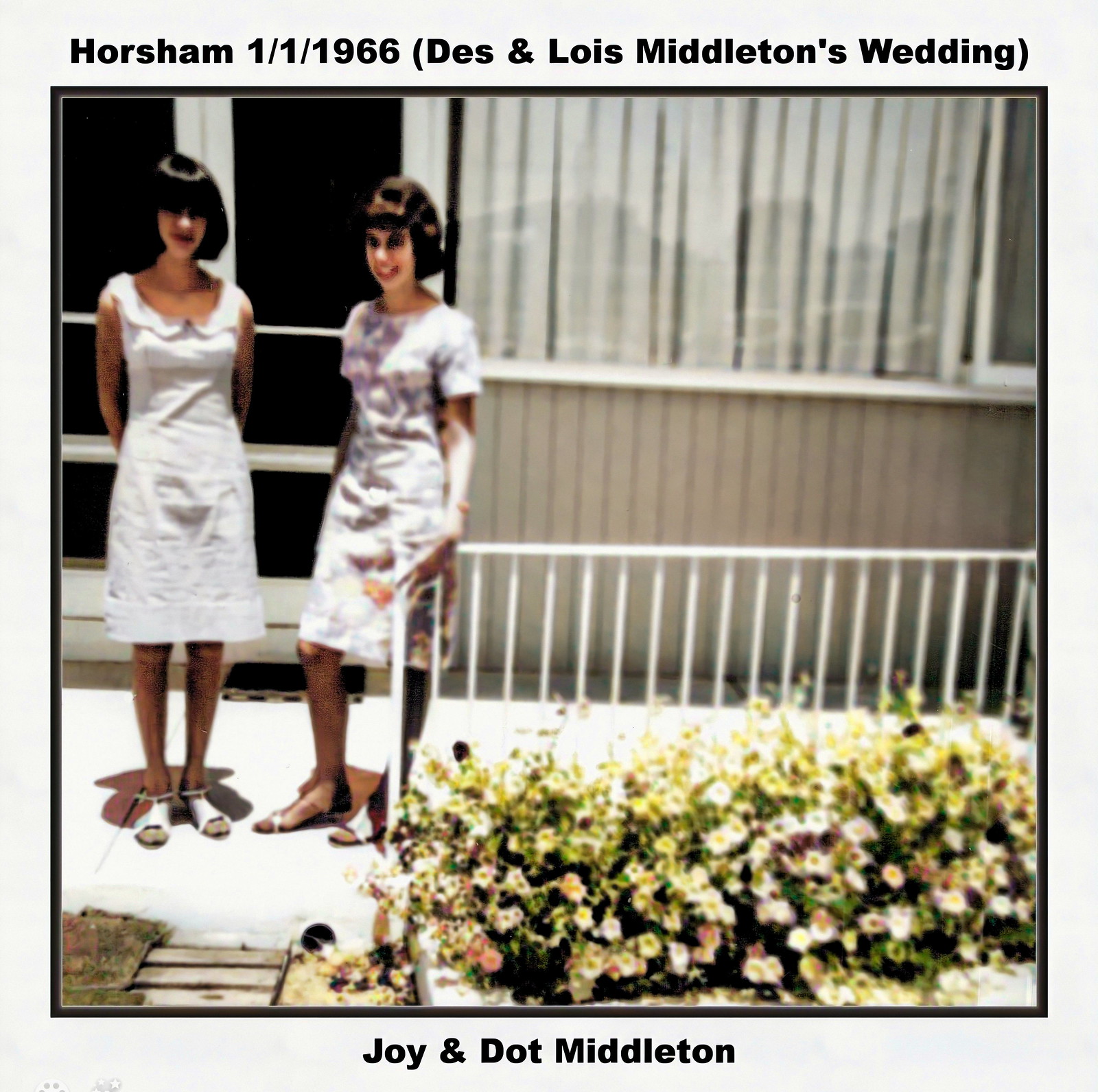In this photograph taken on January 1, 1966, at Des and Lois Middleton's wedding in Horsham, we see two girls, Joy and Dot Middleton, standing outside their home. Both girls have dark bobbed hair. The girl on the left is dressed in a sleeveless white knee-length dress, and the girl on the right is in a white and purple knee-length dress. They are positioned in front of a house with a door and a window featuring vertical white shutters and brown wooden slats beneath. The girl on the left has her hands behind her back, while the girl on the right is gesturing downwards with her left hand. They are standing near a waist-high white metal railing, adjacent to which are some flowering plants. The image is framed with a light blue border, with text inscribed in black letters; the top reads "Horsham, 1/1/1966, Des and Lois Middleton's Wedding" and the bottom reads "Joy and Dot Middleton."